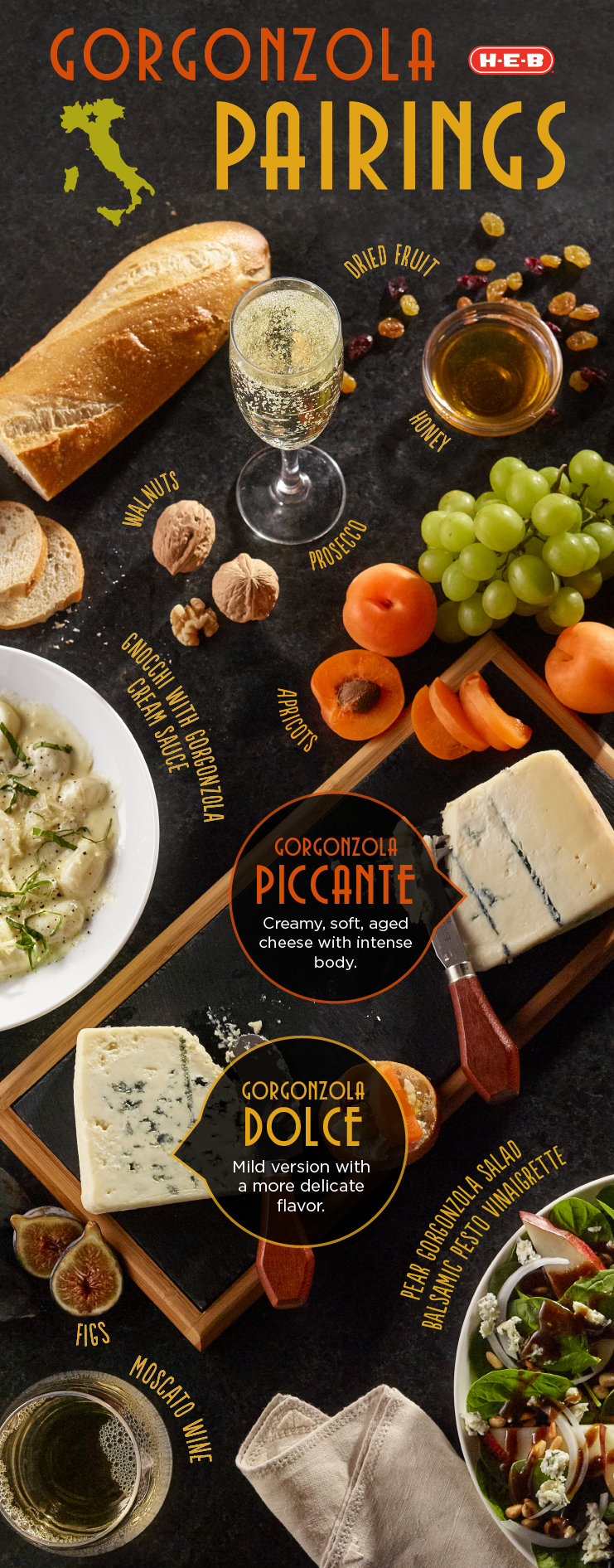This detailed image showcases an advertisement from the supermarket chain H.E.B., promoting "Gorgonzola Pairings." Dominating the top is the title "Gorgonzola Pairings" in vibrant orange and yellow against a black backdrop, with the iconic H.E.B. logo (white letters in a red circle) prominently displayed. The composition resembles an elegant charcuterie board arrangement, featuring a variety of foods perfectly paired with two types of gorgonzola cheese, all labeled for easy identification.

In the center, a brown tray with a black bottom holds two varieties of gorgonzola: **Gorgonzola Picante**, a creamy soft aged cheese with intense body, and **Gorgonzola Dolce**, a milder version with a delicate flavor. The tray also includes an array of accompaniments: slices of French bread, green grapes, and apricots (both whole and diced).

Flanking the tray, the layout extends to display various appetizers and beverages. On one side, a glass of Moscato wine, Prosecco in a champagne flute, and a small jar of honey take their places, each marked by a label. On the other side, we see a delectable pear and gorgonzola salad with balsamic pesto vinaigrette, figs, walnuts, and a pasta dish garnished with gorgonzola cream sauce, possibly gnocchi, all set against the black background, making the colors of the food items pop. A white napkin is neatly placed at the bottom, completing the presentation.

Overall, this enticing display not only highlights the variety of pairings that complement gorgonzola cheese but also serves as a visual guide for creating an impressive spread perfect for any gathering.